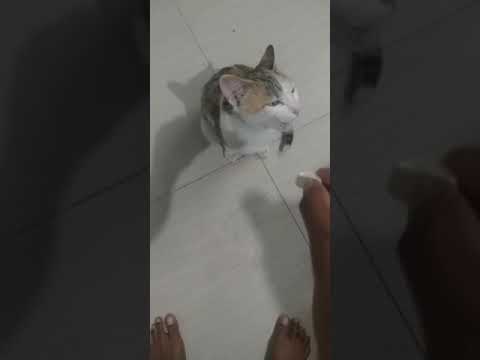The central focus of this image is a multicolored cat with fur in shades of white, brown, tan, gray, and some black, sitting on the ground. The photograph appears to be taken from an upper vantage point, showcasing the cat's indifferent gaze away from a person's hand. The person, who is bare-footed with dark skin, stands on a floor of white tiles. They're holding a small white object, likely a pill or tile, between their index finger and thumb. Surrounding the main image, on both the left and right sides, are vertical strips displaying a close-up and darkened view of the central photograph, as though the image was captured in portrait mode on a cell phone and then adapted for landscape orientation, giving the impression of a still from a video, possibly from platforms like YouTube or TikTok.